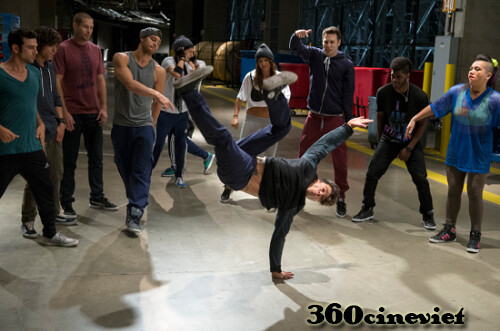In this photograph styled scene, a dynamic moment of breakdancing is captured, possibly set either outdoors on a city street or indoors in a theater, with strong urban vibes. The image showcases a man, suspended mid-air while expertly balanced on his left hand, performing a breakdancing move. He is surrounded by a diverse circle of onlookers, intently focused on his performance.

To the right, moving left, are: a woman in a purple shirt, camel pants, and black sneakers; a black man clad in all black; a white man in a gray hoodie with red pants pointing at the dancer; a woman with a stocking cap, purse, white shirt revealing her midriff, and gray pants; a man in a gray shirt and black pants; another man in a gray tank top also pointing; a man in a tank top and blue jeans with a man in a red t-shirt and black pants behind him; a young man with a hoodie and dark pants; and a final man in a gray v-neck t-shirt and black pants. Each individual is engrossed in the performance, seemingly ready to join in, suggesting they might also be dancers.

Beneath the group, the ground is a hard concrete surface. Despite the ambiguity of whether it’s an outdoor or indoor setting, the surroundings hint at a lively street scene or perhaps an atmospheric warehouse. The bottom right corner of the photograph features the text “360CINEVIET,” adding a distinctive marker to this vivid depiction of street culture.